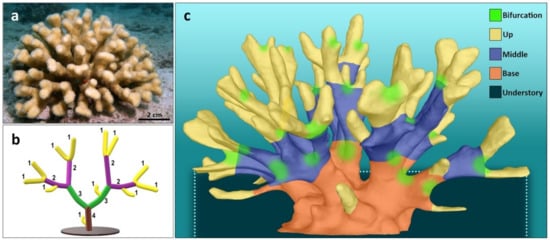The image is a detailed illustration of coral, divided into three sections labeled A, B, and C. Section A, located in the upper left, displays a photograph of whitish coral underwater, with a measurement gauge indicating a length of two centimeters. Section B, directly below A, features a hand-drawn diagram showing the interior structure of the coral, complete with various branches and offshoots, though it's missing a key chart to explain the numbering. Section C, which occupies the majority of the image to the right, is a computer-generated illustration depicting the growth stages of the coral. The color gradient reflects different parts of the coral: the base is a coral peach color, the middle section is blue with purple and green spots, and the topmost section is yellow with green tips. The words "bifurcation," "up," "middle," "base," and "understory" are labeled to help correspond the colors to the various layers of the coral growth.